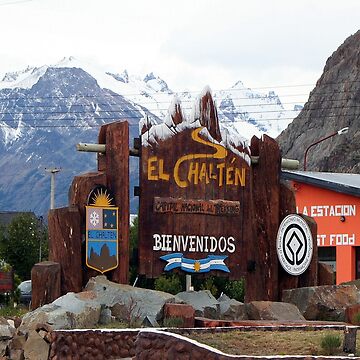The image depicts an outdoor scene during the daytime with a predominantly cloudy sky. In the background, there are majestic mountains, mostly snow-capped, flanking both sides, with one larger mountain on the top right that is not covered in snow. Suspended above are five black electrical wires stretching across the scene. 

Central to the image is a large, dark brown wooden sign that reads "El Chalten," with a blue banner beneath it proclaiming "Bienvenidos." There is a notable orange building with white lettering in the background, accompanied by some trees on the left-hand side. Additionally, a small, official-looking flag, possibly representing a state or country, is visible to the left, adding a touch of regal presence to the image.